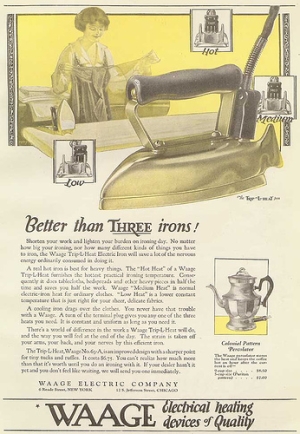This image depicts a vintage advertisement for an electric iron, featuring worn and dull cream-colored paper. Dominating the top half is a yellow rectangle showcasing an illustrated, black-and-white woman with short dark hair, dressed in period attire. She is happily standing behind an ironing board, holding a piece of fabric with an iron placed on the board. Overlaid in front of the ironing board is a prominent image of the iron itself, characterized by a black handle and a gold or bronze body. The ad prominently states, "Better Than Three Irons!" in bold black font, with "three" underlined. Below this claim, five paragraphs of small, unreadable text are present. Positioned to the right side within a small rectangle, there's a silver picture of what seems to be a chrome electrical teapot with a black handle. The bottom of the ad declares, "WAAGE Electrical Heating Devices of Quality." Additionally, the iron's various settings—low, medium, and hot—are indicated by logos.